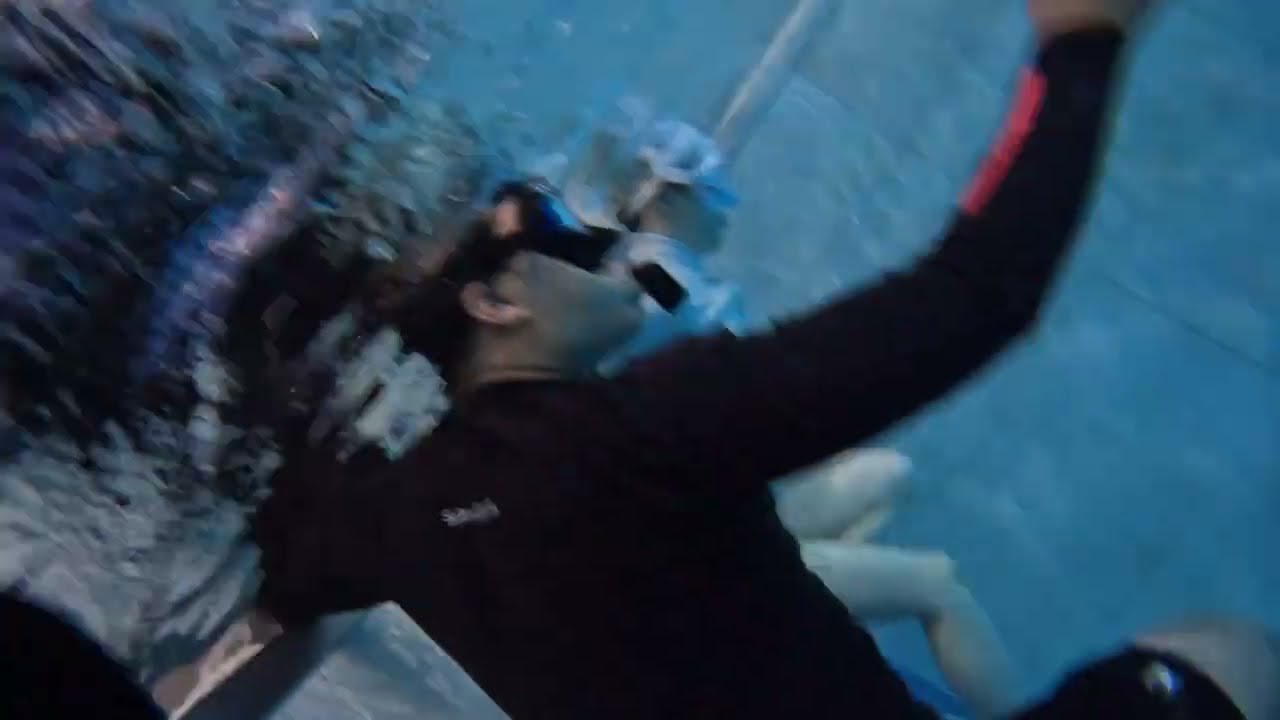An underwater photograph captures an intimate, slightly angled view beneath the water's surface, which is visible in the top left corner. Two individuals are partially submerged, their heads poking out of the water. The person in the foreground wears a black long-sleeved shirt adorned with red squares at the cuffs, black shorts, and a pair of black-rimmed goggles attached to a black snorkel. White lettering can be seen on the back of their shirt. This person has short grayish hair and their right arm is raised, as though they are taking a selfie, and they are gazing towards their hand. Behind them floats another person, clad in a white bathing suit and white-rimmed goggles with a white snorkel, sitting or lying against the far dark gray pool wall, which carries a slight blue tint from the water. The image is somewhat blurry, hinting at a possible low resolution or high compression, which adds to the mysterious underwater ambiance.